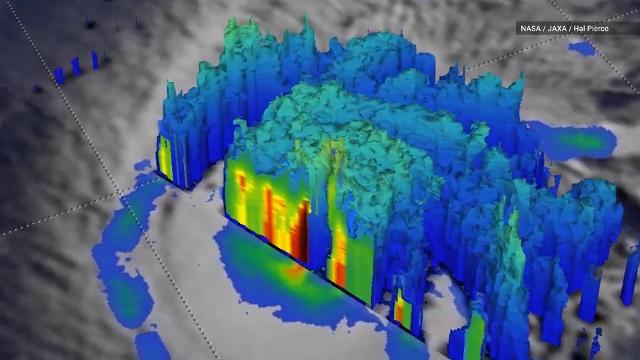This detailed image, presented by NASA/JAXA/Hal Pierce, is a satellite photo depicting a fierce storm, possibly a hurricane, characterized by a swirling mass of storm clouds. The base layer of the image is in black and white cartography, showcasing a landscape orientation. At the center of the storm lies a distinctive blue and green area surrounded by intense colorations of yellow, orange, and dark red, suggesting varying intensities and heights of cloud tops. The outer gray perimeter transitions into white circulating bands of clouds. A black horizontal rectangle in the top right corner bears white text indicating its source. The detailed blowout diagram over the hurricane’s center highlights the storm's structure and severity, augmented by color illustration to indicate different cloud heights and formations. The overall effect is a vivid representation of the storm's power and the intricate weather patterns being tracked.